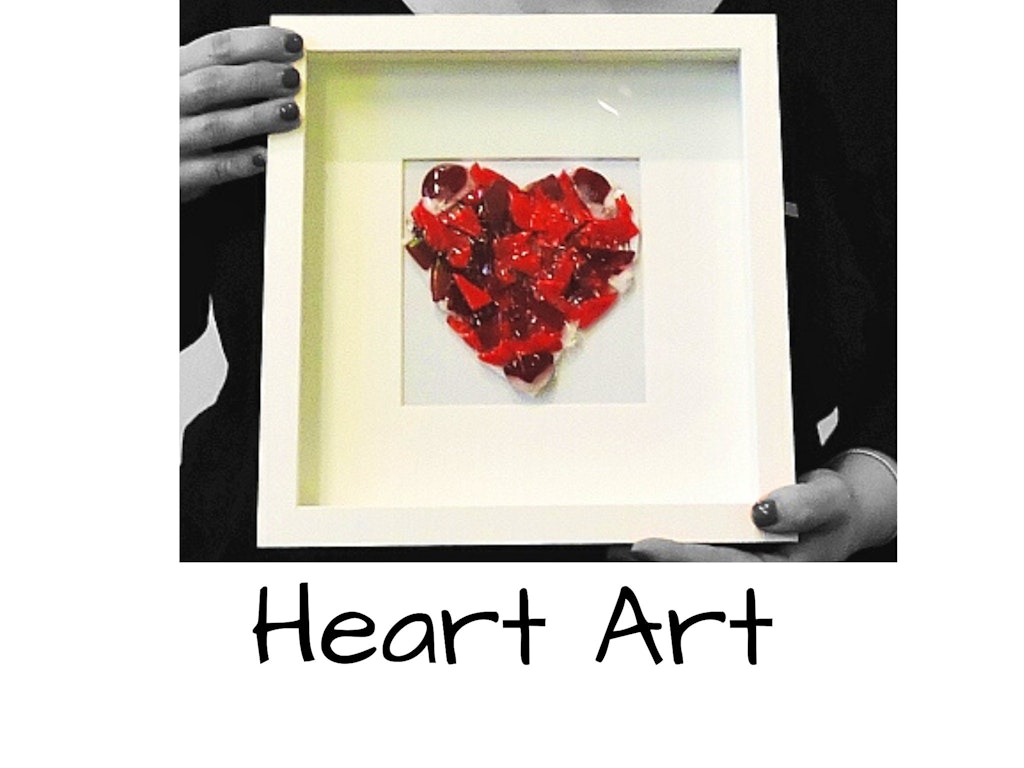The image titled "Heart Art" is an intricately detailed black-and-white photograph with selective color elements. It features a person, dressed in black clothing and adorned with dark nail polish, holding a white shadow box frame with a wide cream mat. The person wears a thin, light-colored bracelet on their left wrist. The setting is primarily monochromatic, focusing on the individual's hands—right hand gripping the upper left corner and left hand holding the lower right corner of the frame. 

Inside the shadow box, a vivid, vibrant heart stands out, crafted from shiny, broken shards of material. These shards vary in color from bright blood red to maroon, and even to a deep red verging on black, with occasional white accents interspersed. The contrast between the colorful heart and the grayscale photograph creates a striking visual effect. Below the heart, "Heart Art" is inscribed in black text, melding photographic realism with graphic design elements.